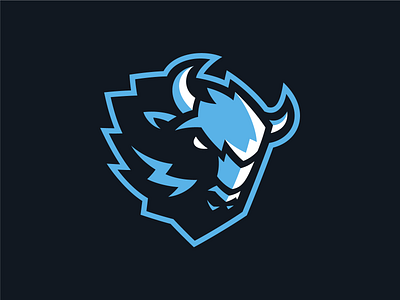This is a detailed drawing of a bull or possibly a buffalo head, featuring an aggressive stance that suggests it might serve as a sports team mascot. The image is set against a dark background, which is either black or a very dark navy blue. The face of the animal is predominantly colored in vibrant blue, black, and white, giving it a striking and dynamic appearance. The eyes are white, with visible black nostrils, and the entire head is composed of sharp, angular lines that create a squared-off look. Distinctive features include two prominent horns and a blue lightning bolt towards the bottom left of the face. The image has a computer-generated feel and is printed in such a way that it could easily be featured on a sports jersey or a hat. This combination of colors and shading effects highlights the fur and gives a sense of motion and intensity, with the head slightly tipped downwards, eyes peering through the top of its head, enhancing its fierce and determined expression.